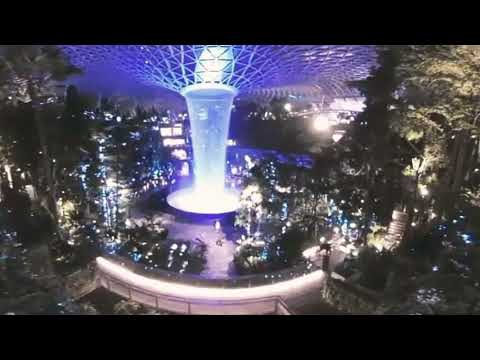The image captures a slightly distorted yet iconic view of the Jewel Changi Airport's Rain Vortex in Singapore. Dominating the center is a brilliantly lit, cylindrical waterfall feature that rises from a circular pool in the ground, opening up into a ceiling structure characterized by grid-like netting. This futuristic, blue-tinged architectural marvel is surrounded by lush green trees and bushes adorned with numerous twinkling lights, creating an otherworldly ambiance. To the left and right, rows of illuminated trees flank the central attraction. In the foreground, a guardrail delineates a pathway or observation deck where a few individuals can be seen walking. The image is bordered by thick black margins at the top and bottom, adding to its dramatic presentation.